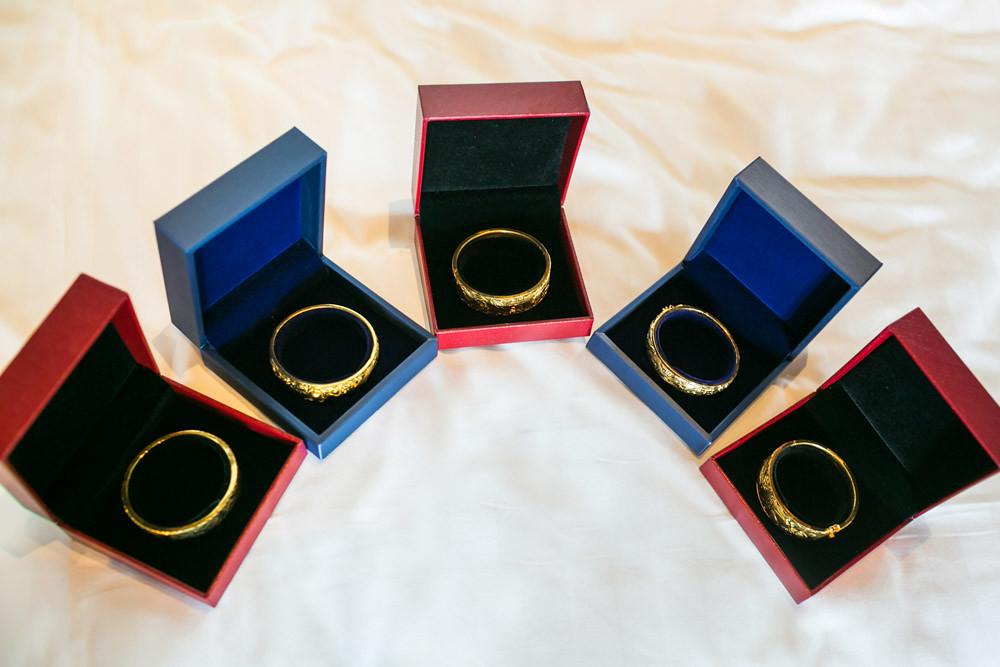This photograph features five jewelry boxes arranged in a semicircle on a white, silky fabric that has a slight orange tint due to the lighting. The boxes alternate colors in a red-blue-red-blue-red sequence. Each box contains an identical, gold-colored ring that is round, flat, and ornately decorated. Inside the boxes, there is a black insert, possibly made of fabric, providing a contrasting background for the rings. The overall presentation highlights the luxurious feel of the set with its silk-like backdrop and the striking contrast between the colorful boxes and the black fabric interior.